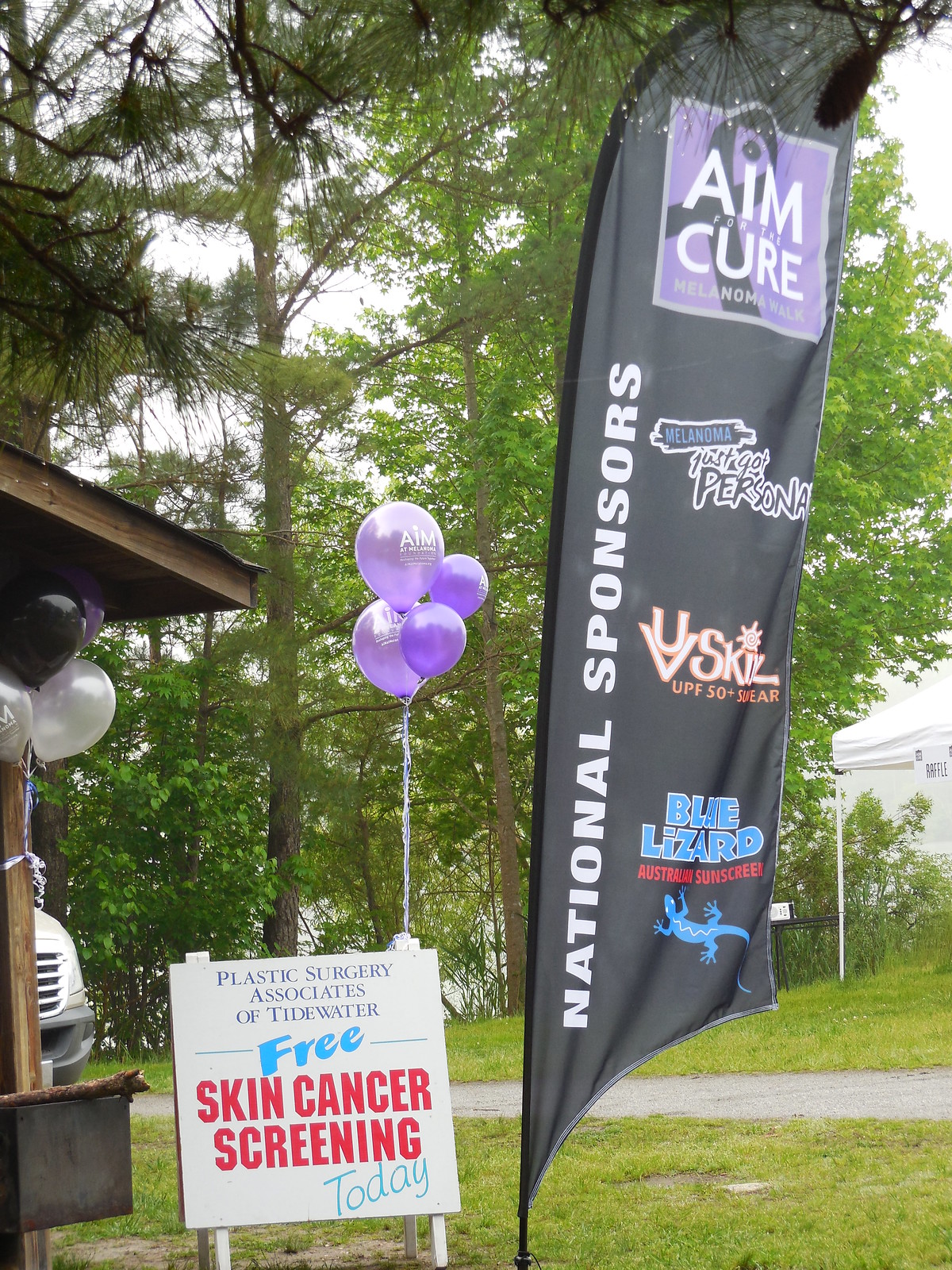The image captures an outdoor event at what appears to be a county fair. Central to the scene is a tall, black banner flag on the right, which reads "National Sponsors" in white text along the left side. The right side of the flag displays sponsor logos such as Blue Lizard Australian Sunscreen and others. To the left of the banner flag is a small, collapsible wooden sign promoting free skin cancer screenings by "Plastic Surgery Associates of Tidewater." The sign features the words "Free" and "Today" in light blue and "Skin Cancer Screening" in bold red text. Attached to the sign are four purple balloons with the logo "Aim at Melanoma." The setting appears overcast, with several trees in the background and a walkway that invites fairgoers to stop by the booth. Nearby, a white tent structure and the awning of a building frame the left and right edges of the photo, respectively, completing the picturesque view of this healthcare initiative amidst a lively outdoor environment.